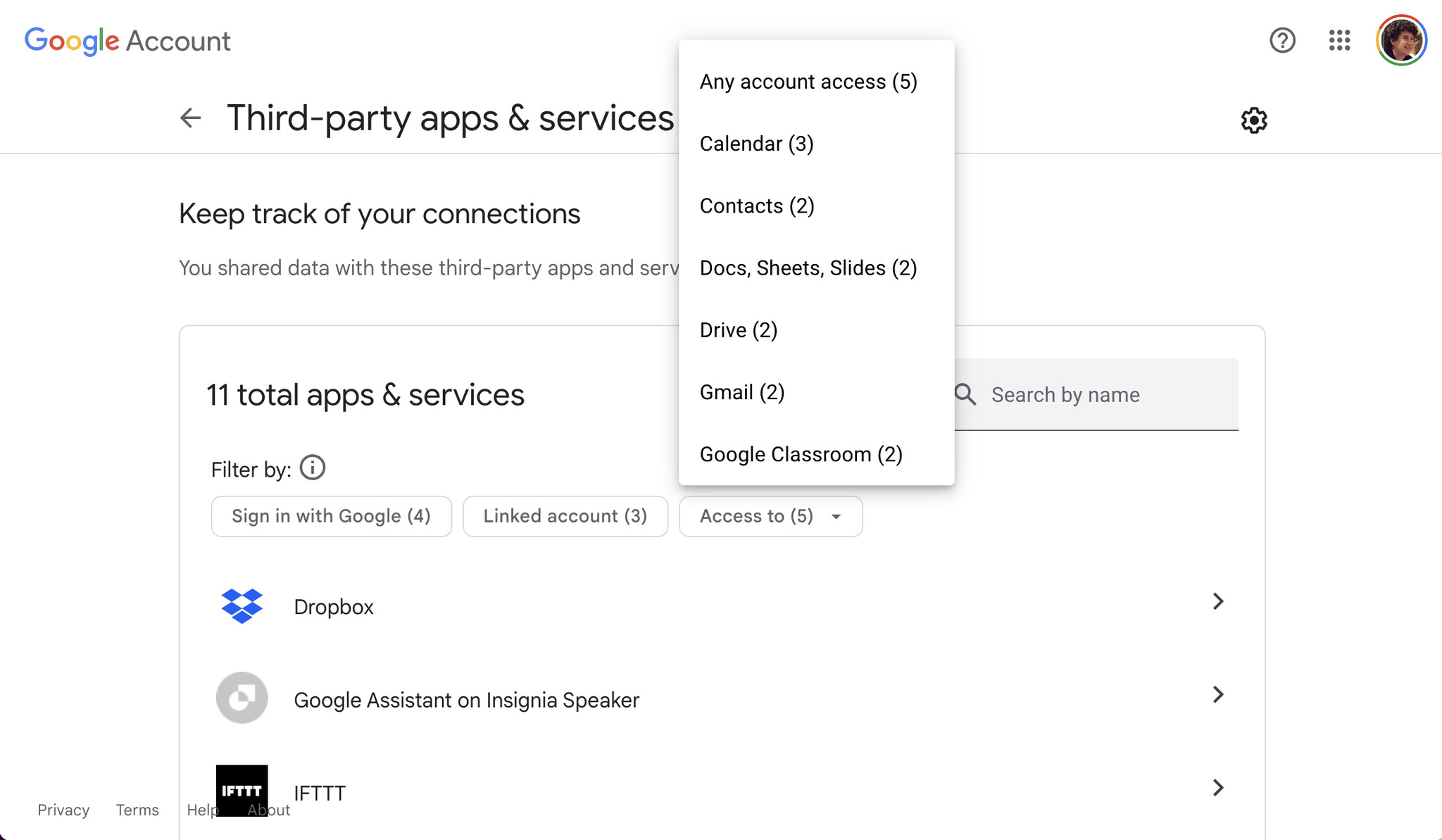Here is a cleaned-up and detailed caption for the image:

---

This image captures the Google Account settings page of a user. The background is predominantly white, creating a clean and simple interface. At the top left corner is the iconic Google logo, displaying its signature colors of blue, red, yellow, and green. Adjacent to the logo is the word "Account." Over at the top right corner, there are two icons: a "Help" button and the user’s profile picture.

Below the Google logo on the left side, there is a back arrow accompanied by the text "Third-party apps and services." Underneath, there is a section with a descriptive message: "Keep track of your connections. You share data with these third-party apps and services," followed by a count indicating "11 total apps and services." This section provides users with the ability to view and manage which third-party applications have access to their data.

Prominently, a dialog box appears in the middle of the screen, listing the specific access levels and apps: 
- "5 Calendar"
- "3 Contacts"
- "2 Docs, Sheets, and Slides"
- "2 Drive"
- "2 Gmail"
- "2 Google Classroom"

Additionally, at the bottom of this dialog box, specific third-party services such as "Dropbox," "Google Assistant on an Insignia speaker," and "IFTTT" are mentioned, indicating connections with these services.

---